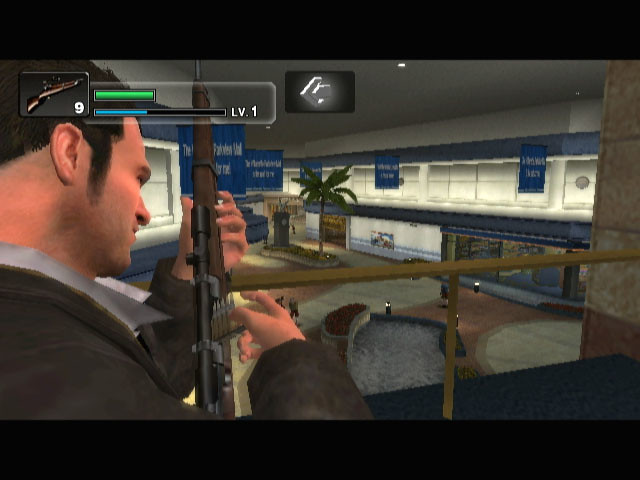The image is a horizontal rectangular screenshot from an older video game, featuring a male figure on the left side in the foreground. The man, possibly an AI character, has short brown hair, long sideburns, and is dressed in a black jacket over a blue shirt with a white collar. Both of his hands are on a lengthy dark brown rifle with a black scope, seemingly captured in the moment of reloading it. An icon of the rifle with the number 9 beside it is present in the upper left corner, accompanied by a graph showing a medium-long green line and a partially filled blue line labeled "LV-1."

The setting appears to be the interior of a mall, observed from an elevated position. The background features a gold railing stretching horizontally and a mixture of tan and orange tiles on the floor below. There's also a tall palm tree centrally located, surrounded by blue rectangular banners. The room has a white ceiling dominating the upper half, and the area below seems to be illuminated but blurry, with possible shops scattered around. The general ambiance of the game suggests an Electronic Arts title, and the overall image is slightly pixelated, indicating its age.